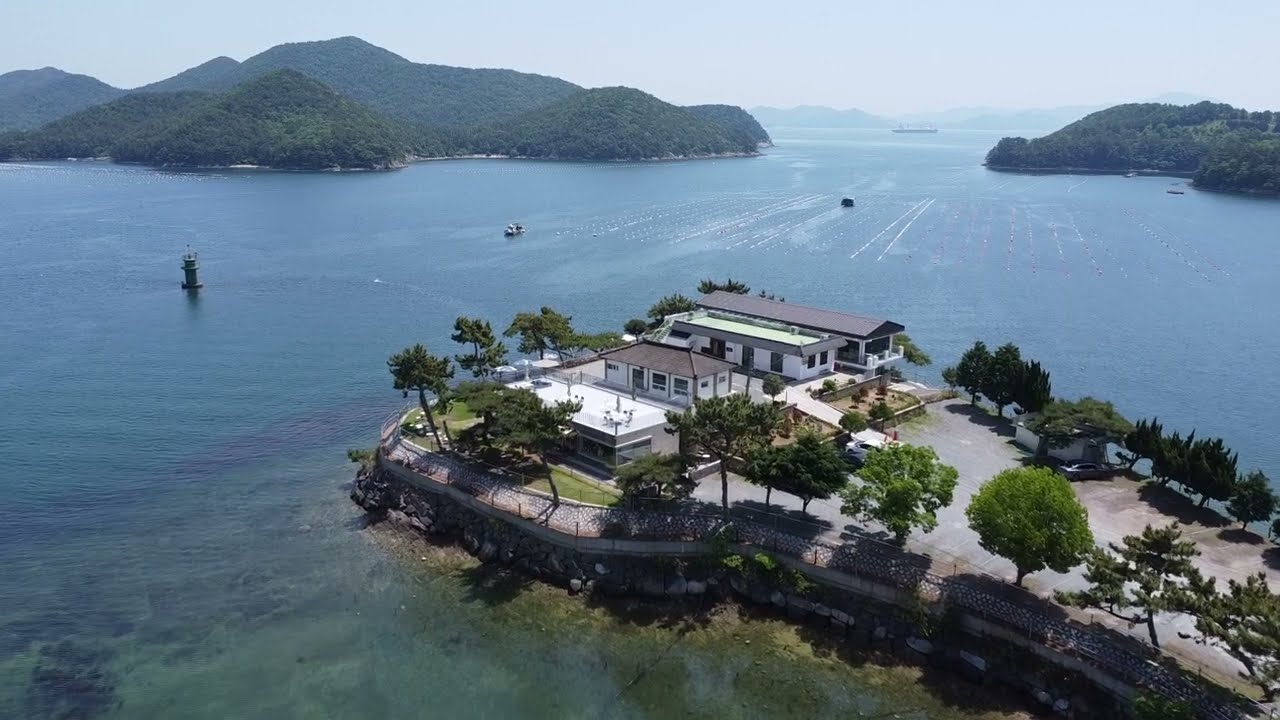An aerial drone shot captures a picturesque island surrounded by a calm body of water. Dominating the island is a sprawling white mansion with brown roofs, resembling a luxurious beach villa, complete with its own private road and parking area. This grand house occupies much of the island's area, with concrete driveways and clusters of trees adding to its charm. Adjacent to the island, the water hosts a large, gray, metallic buoy on the left side of the frame and various boats, including a very large one, miles away in the distance. The background reveals an overcast, cloudy sky and verdant hills blanketed with thick, green trees, stretching from the far left to the right, hinting at the edges of other islands. The shallow waters around the island suggest that one might easily wade near the shore, enhancing the serene, vacation-like atmosphere of this idyllic retreat.